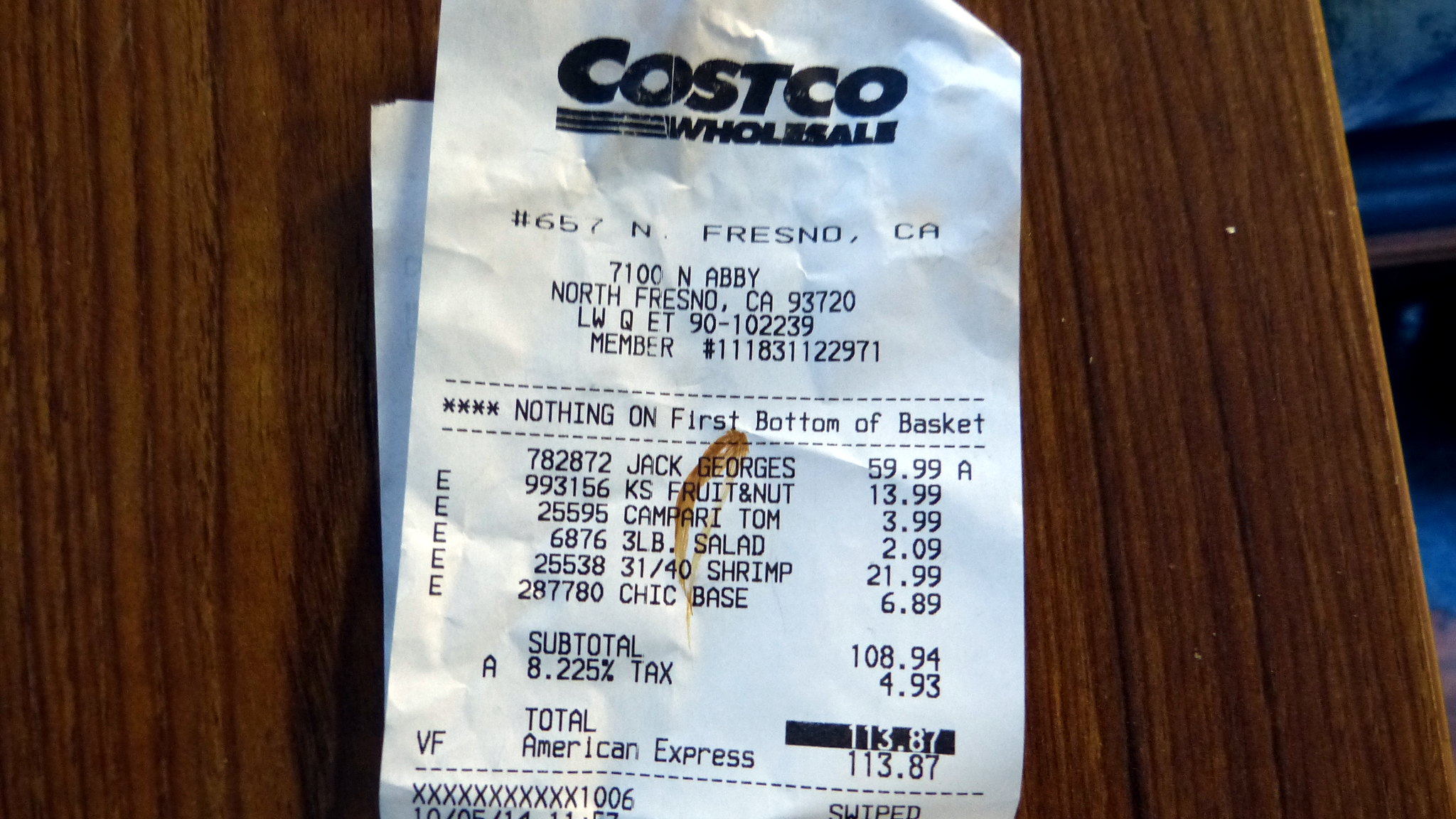A detailed caption for the image is as follows:

"A white receipt from Costco, featuring black lettering, is placed on what appears to be a brown wooden desk. At the top of the receipt, 'Costco Wholesale' is prominently printed in bold letters alongside the recognizable Costco symbol. The receipt, smudged with an unidentified brown mark, lists several purchased items, including fruit nuts, a three-pound salad, and 31/40 shrimp. The total amount for the purchases is $108.94, with an additional tax of $4.96, summing up to a final charge of $113.87. The payment was made using an American Express card. The receipt also includes a reference to Costco's Fresno, California, location with the address details 'Dollar Sign 657, 7100 Aberry, North Fresno, California,' and a Member ID number."